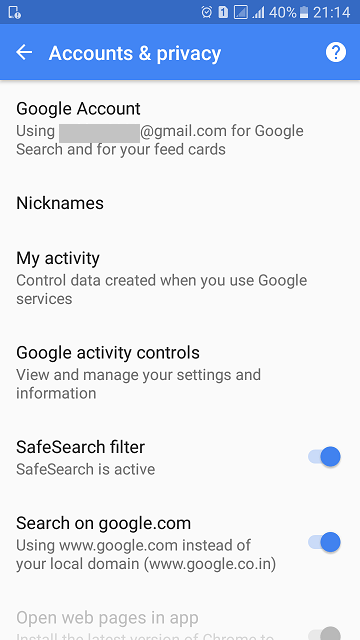The image displays a Google settings page, starting from the top left with the headings "Accounts and Privacy." In the top right corner, the screen shows a battery level at 40% and the time as 21:14. Below a prominent blue banner, there's a section titled "Google Account," with an obscured username, formatted as "username@gmail.com."

Scrolling further down, the page features various sections including "Search" and "Your Feed Cards," followed by sub-sections such as "Nicknames," "My Activity," and "Control Data Created When You Use Google Services." Additionally, there are "Google Activity Controls," "View and Manage Your Settings and Information," and "SafeSearch Filter," indicating that SafeSearch is active.

On the right side of these options, a blue button signals the selected choice. From left to right, another option reads "Search on google.com" with "www.google.com" instead of "www.google.co.in" (noted in parentheses), also marked with a blue selection button.

The final visible option is "Open Web Pages in App," where the associated selector button is gray, indicating it is not activated. There is further text below this, but it is obscured and not readable in the image.